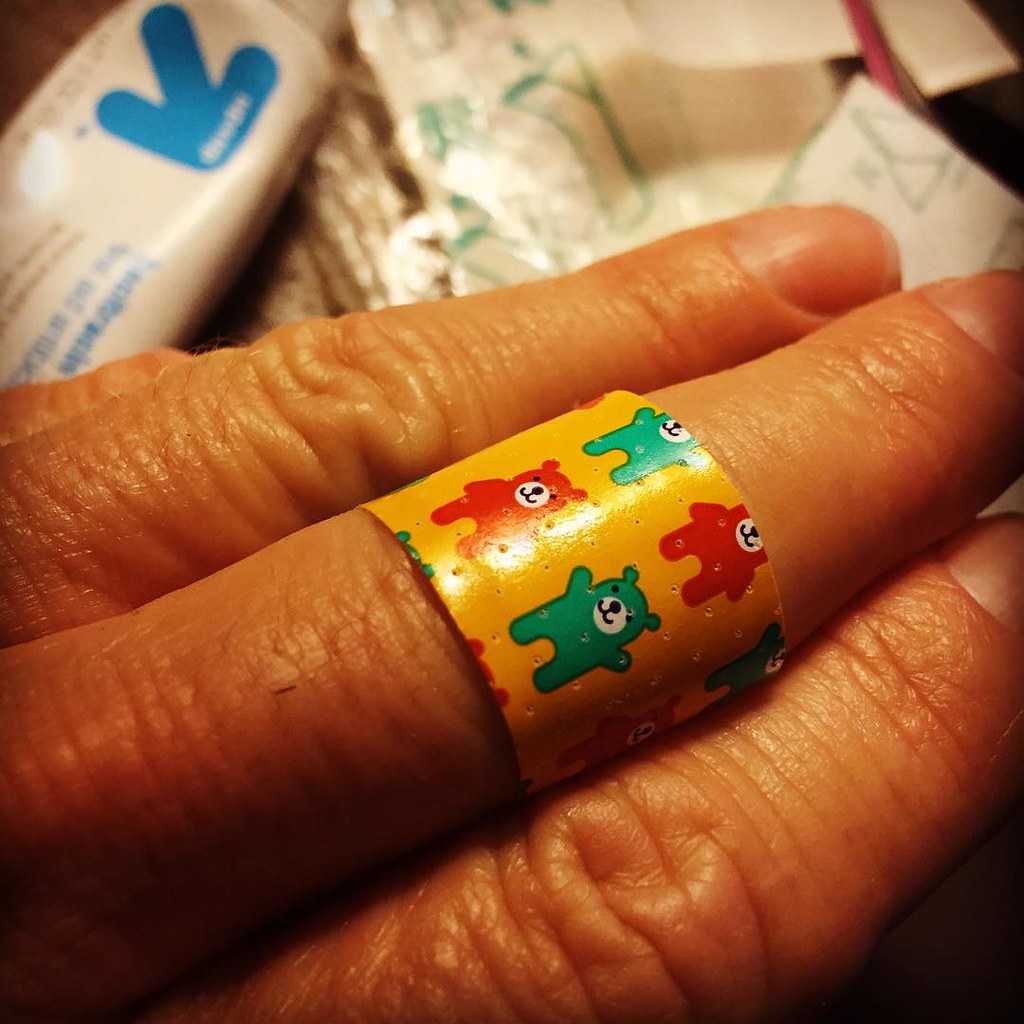This image is a detailed close-up of an elderly Caucasian woman's hand, which appears wrinkled and aged, possibly around 60 or 70 years old. The hand is central in the frame and occupies nearly half of the image, with short unpolished nails and a distinctive children's band-aid wrapped around the middle finger. The band-aid is yellow and adorned with cartoon bears in red, green, and cyan, giving it a whimsical appearance. The background, although somewhat blurry, suggests an indoor setting, potentially a bathroom, with visible items such as a tube of cream, wet wipes, and possibly diapers. Various colors like tan, orange, red, white, black, green, blue, and brown can be spotted in the scene. The light source illuminates the objects, highlighting a blue arrow on the packaging near the upper left-hand corner.